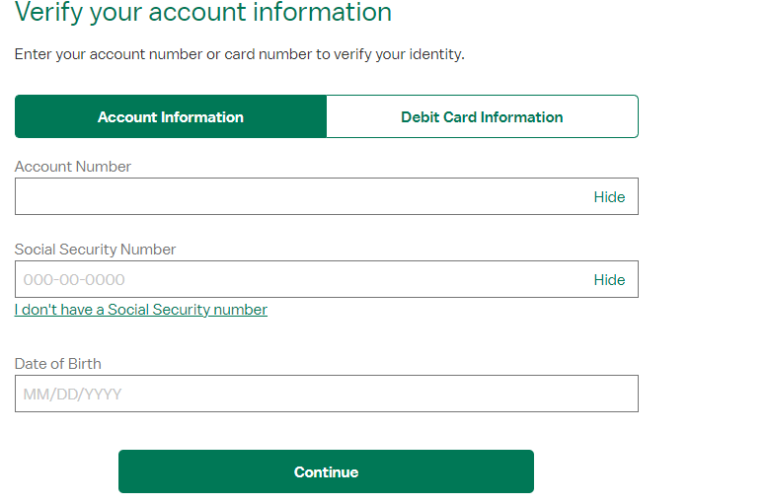The website's interface prominently displays a large green heading that reads, "Verify Your Account." Below this, smaller text instructs users to "Enter your account number or card number to verify your identity." 

The page features several sections differentiated by color:

1. **Account Information Section**: 
    - **Green Bar**: This bar is labeled "Account Information" and is attached to a white bar labeled "Debit Card Information."
    - **Account Number Entry**: A white input field labeled "Account Number" includes a green "Hide" option on the right side.
    - **Social Security Number Entry**: Below the account number field, users are prompted to add their Social Security Number with another "Hide" option in green on the right. Additionally, there's clickable green text stating, "I don't have a social security number."

2. **Date of Birth Entry**:
    - A designated area for entering the date of birth requires input in the format MM/DD/YYYY, with separate fields for month, day, and year.

At the bottom of the form, a prominent green bar with white text in the center says "Continue." The overall design features a clean white background, with the predominant colors being green for headings, bars, and clickable options.

Overall, the user interface is clear and emphasizes verification steps with distinctive green highlights to guide the user through the process.